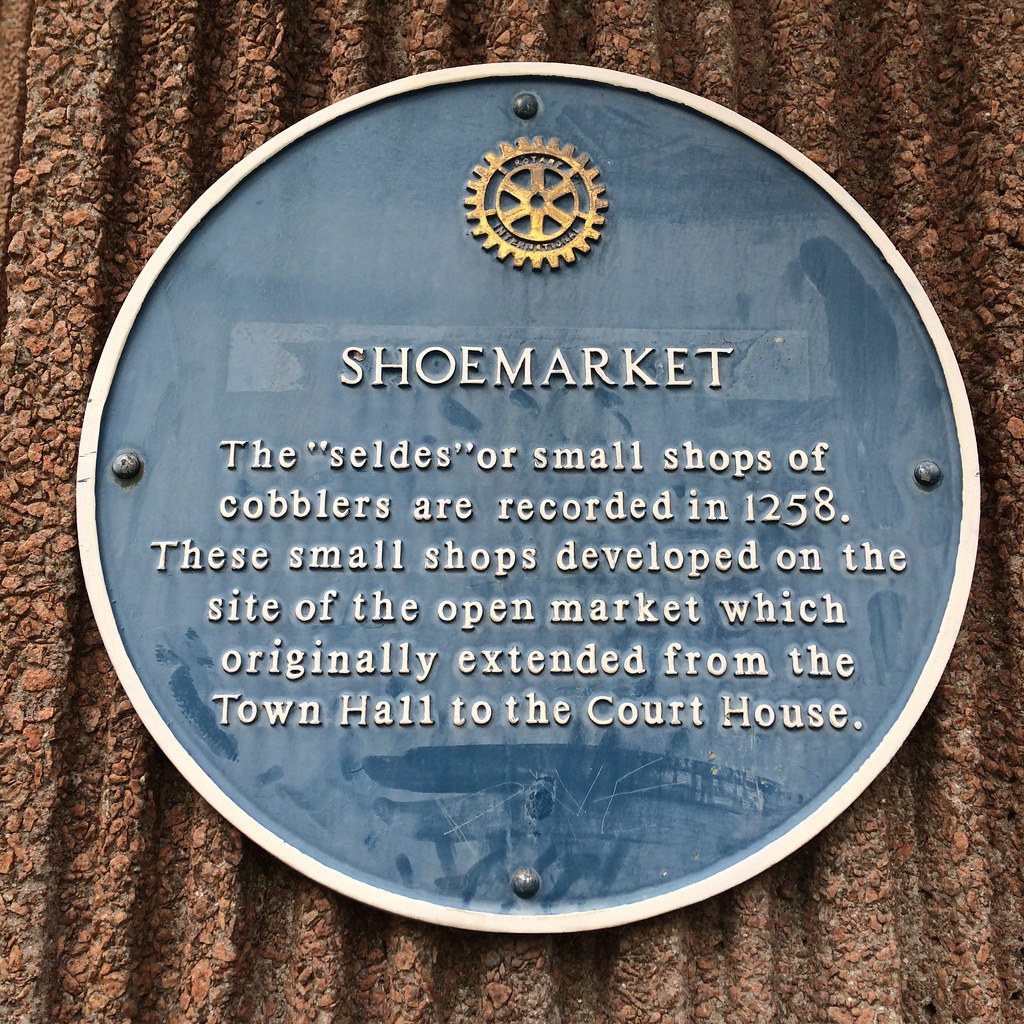The photograph features a circular blue plaque with a gold Rotary International logo at the top, bearing a silver metallic border around the emblem. The text, embossed in white, reads: "Shoe Market. The small shops of cobblers, or 'seldas,' are recorded in 1258. These small shops developed on the site of the open market, which originally extended from the town hall to the courthouse." The plaque is affixed to what appears to be a stone or concrete wall with a rough, textured surface. The background, varying in shades of light red or gray, highlights the historical significance of the site where cobbler shops once flourished. The plaque stands out centrally in the image, symbolizing a tribute to the area's rich artisanal heritage.